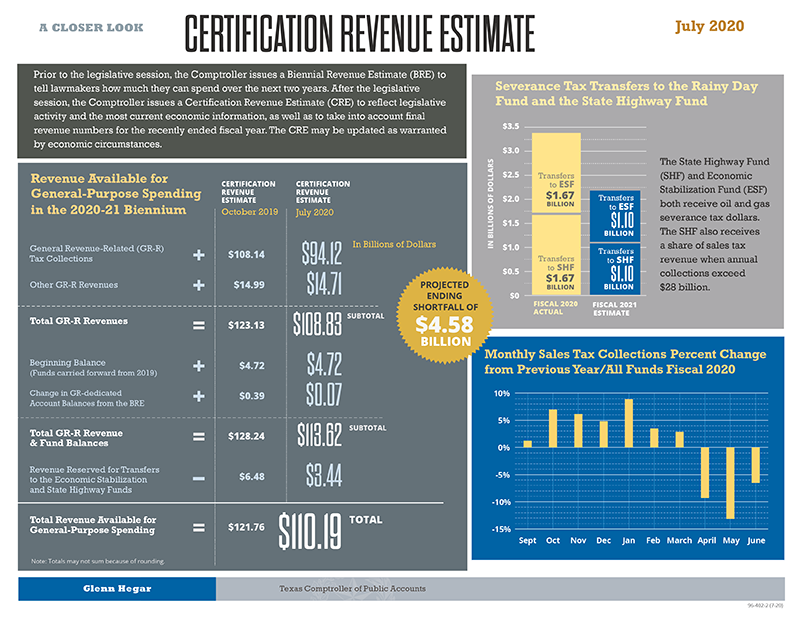**Infographic Caption: Certification Revenue Estimate - A Detailed Breakdown**

This informative infographic titled "Certification Revenue Estimate" is presented with a bold, block-like black header. In the top-left corner, under the smaller font heading "A Closer Look," and dated "July 2020" in a gold-colored font located at the top right, the infographic is organized into four distinct quadrants.

1. **Top Left Quadrant:**
   - **Description:** A dark gray rectangular section.
   - **Content:** Contains detailed information in white text about the Certification Revenue Estimate (CRE) and legislative activities.

2. **Top Right Quadrant:**
   - **Description:** A light gray infographic section.
   - **Content:** Features a bar diagram titled "Severance Tax Transfers to the Rainy Day Fund and the State Highway Fund" in yellow text. The bar diagram is positioned on the left, with an adjacent black text block on the right detailing the State Highway Fund and the Economic Stabilization Fund, presumably in a comparative analysis format.

3. **Bottom Left Quadrant:**
   - **Description:** The largest section of the diagram, a dark gray chart.
   - **Content:** Displays various spending figures concluding with a total at the bottom. The chart is titled "Revenue Available for General Purpose Spending in the 20-21 Biennium" using a gold font.

4. **Bottom Right Quadrant:**
   - **Description:** A blue section.
   - **Content:** Contains a bar graph titled "Monthly Sales Tax Collection Percent Change from Previous Year All Funds Fiscal 2020." The graph visually represents months and their respective percentage changes.

**Central Highlight:** A prominent gold circle at the center of the diagram emphasizes the "Projected Ending Shortfall of $4.58 Billion."

**Authorship and Authority:** At the very bottom of the infographic, outside the main visual elements, the names "Glenn Hegar" and "Texas Comptroller of Public Accounts" are distinctly mentioned, attributing the source and authority behind the information presented.